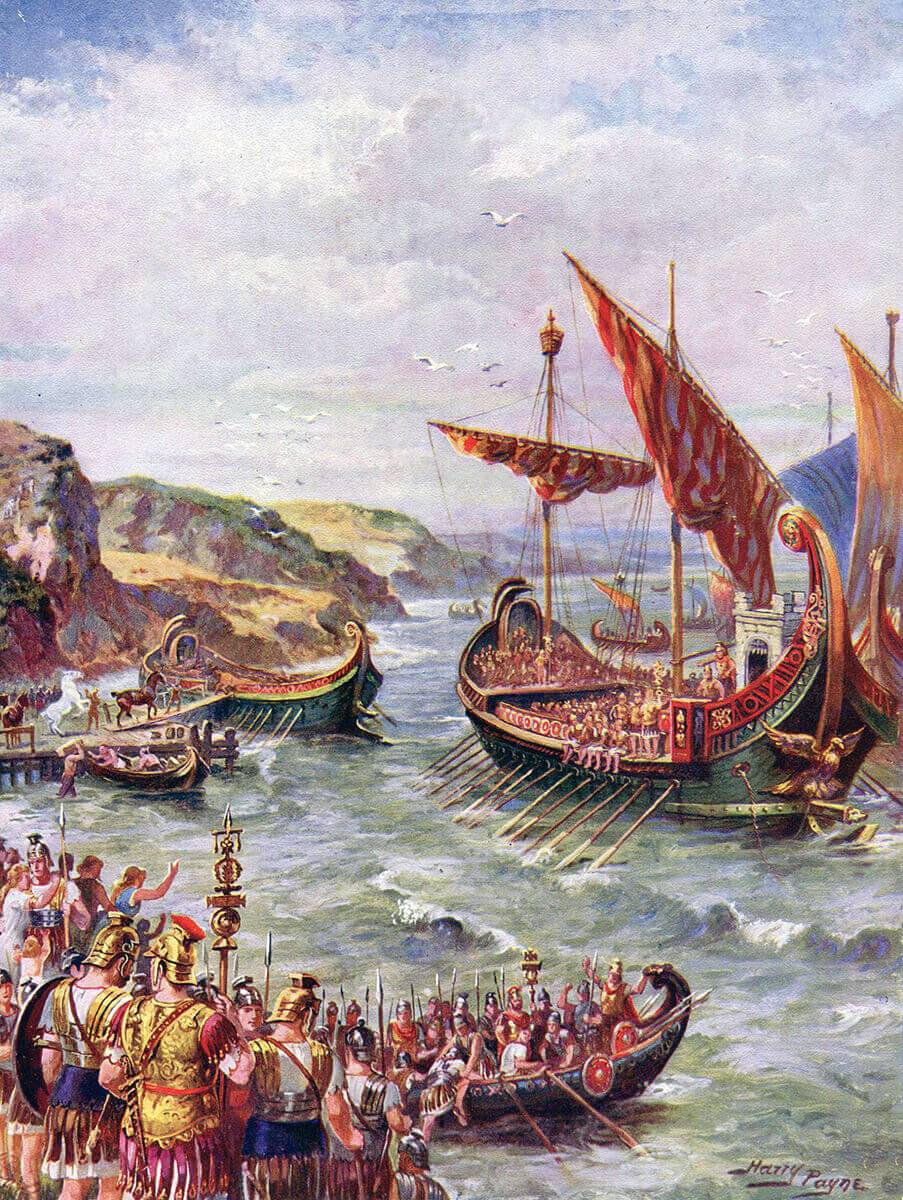This painting, likely depicting a scene from antiquity, features highly detailed elements both on land and sea. Dominating the visual narrative is a prominent ship, painted with a green hull and adorned with multiple flags, situated close to a rocky shore. This vessel is equipped with two masts that hold rolled sails and a string of oars extending from its center, suggesting readiness for rowing. In the foreground, on the bottom left, a group of ancient warrior figures wearing gold-colored, crested helmets stand poised near a cliff edge. These soldiers, clad in shiny armor and brandishing circular shields and spears, bear a strong resemblance to Roman or Spartan warriors.

To the left side of the painting, the edge of the water where the soldiers stand is visible. Near them is another smaller boat, also equipped with oars and occupied by men carrying red shields. The waters beneath these boats are depicted with realistic waves and white spray, capturing the dynamic movement. Above, a cloudy blue sky filled with white and gray clouds stretches across the scene, populated by flying seagulls.

The background features cliff-laden, rocky shores adding to the dramatic landscape. A medium-sized boat appears to be in preparation, possibly being loaded with supplies or horses. This complexity of maritime and terrestrial elements is rendered meticulously, echoing the styles from possibly the 10th or 11th century. The painting is signed "Harry Payne" in the bottom right corner, grounding the artwork in a specific historical and artistic context.